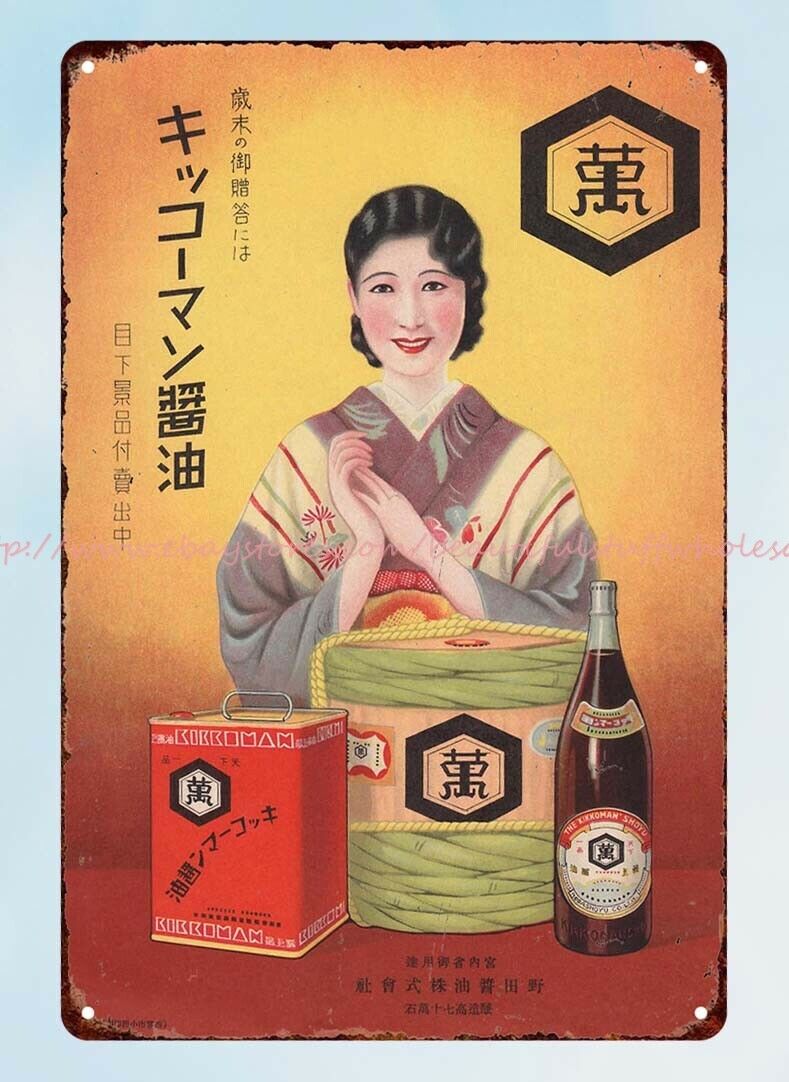This rectangular image, approximately six inches tall and four inches wide, is framed by a gradient light blue border that darkens towards the top. A pale pink cursive text crosses the image horizontally, though it is indistinct. Central to the blue border is a beveled rectangular area transitioning from a light yellow at the top to a deep orange at the bottom, punctuated by small holes at each corner.

The central artwork features an illustration of an Asian woman with curled black hair, pale white skin, rosy cheeks, and red lips. She is smiling and clasping her hands to the left. She is adorned in a traditional kimono-like garment, patterned with muted purple, yellow, and blue hues, accented by bright red lines and floral designs, and touches of gray-green.

Positioned before her are three items: a red canister with a handle, possibly a condiment container, a central cylindrical bundle wrapped with yellow and green ropes, and a bottle on the right resembling soy sauce. All three items are marked with foreign text, likely Japanese. Additional Japanese characters appear on the left of the rectangle, and a brand icon occupies the upper right corner of the image. This image seems to be an advertisement, probably for traditional Asian condiments.